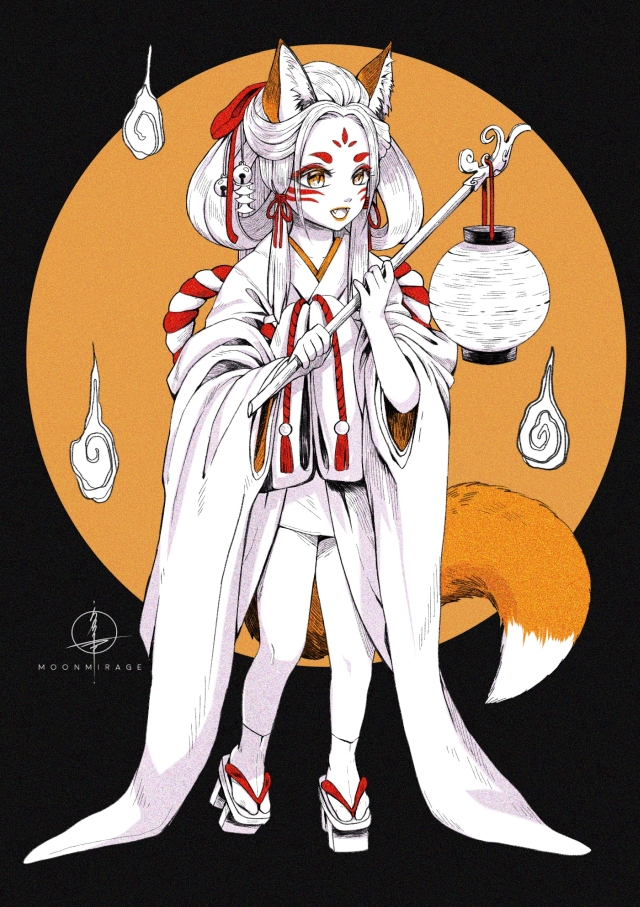This image is a detailed anime illustration featuring a female character with fox-like traits, set against a black background with a prominent orange circle. The girl stands in front of the circle, showcasing orange fox ears lined with white fur and brown on the outside. She has long, blonde or white hair intricately looped and tied back with a red bow, adorned with bells and possibly a pagoda decoration. Her face is marked with three orange symbols on her forehead, red fleur-de-lis designs, and orange swashes underneath her golden eyes. She wears a long white robe with red accents, which touches the ground, and thong sandals with red straps. A bushy fox tail wraps around and points down behind her. In her arms, she holds a scepter, from which hangs a round lantern with a red hook. Surrounding her are droplets and swirly designs, adding a mystical aura to the image. The text "Moon Mirage" along with a logo is also present on the photograph.